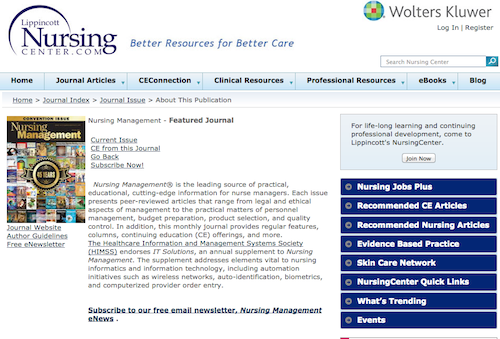The Lippincott Nursing Center website, accessible at LippincottNursingCenter.com, offers a variety of resources under the tagline "Better Resources for Better Care." At the top right corner, the site features options to log in or register, accompanied by a search bar positioned just below. A horizontal blue navigation bar spans across the page, divided into sections labeled Home, Journal Articles, CE Connection, Clinical Resources, Professional Resources, E-books, and Blog.

To the left side of the page, there is an image of the cover of the Nursing Management journal, which features a collage of pictures. Situated in the middle, a section titled "Nursing Management Feature Journal" highlights the current issue, followed by a detailed explanatory paragraph. Within this paragraph, bold text invites visitors to subscribe to a free email newsletter called Nursing Management e-News.

On the right side of the main content, there is a vertical column of blue boxes stacked one above the other, each containing different options and links for further navigation.